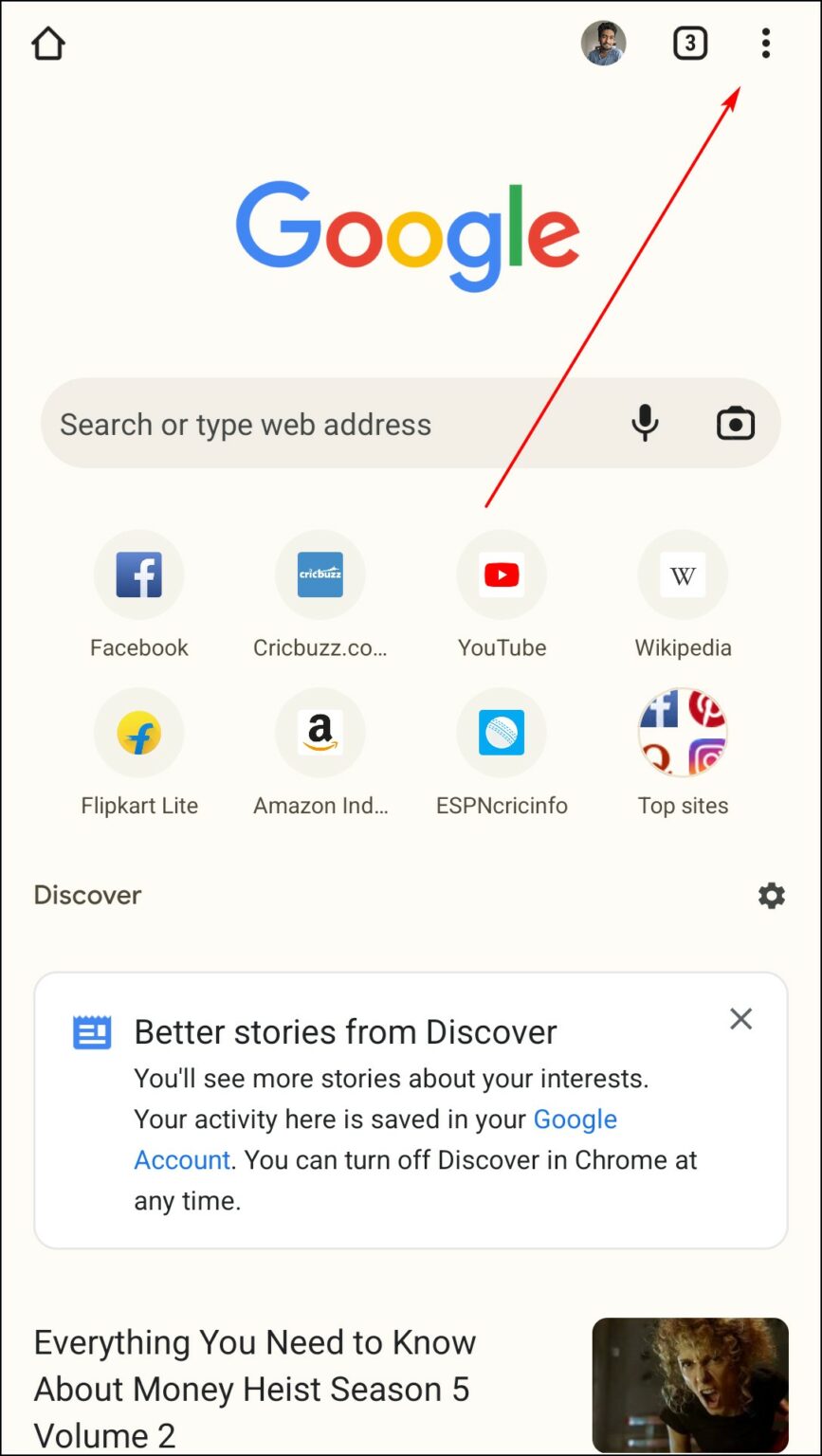The image captures a screen from a mobile phone showcasing a Google search page. Dominating the screen is the word "Google" in its classic, colorful logo featuring a blue "G," a red "o," a yellow "o," a blue "g," a green "l," and a red "e." Beneath the logo is a prominent search bar awaiting input.

At the top-left corner of the screen is a home button, an atypical placement for such an icon. To the right of the Google logo, an icon depicting a person—likely an Indian male in his thirties—suggesting the phone owner’s profile is visible. The browser interface shows that three tabs are open, with a vertical ellipsis (three dots) located in the top-right corner next to these tabs. A red line with an arrow points to these three dots, drawing attention to them from just beneath the web address bar.

Just below the web address bar, a collection of frequently visited sites is displayed. These include icons for Facebook, Cricbuzz, YouTube, Wikipedia, Flipkart Lite, Amazon India, ESPN Cricinfo, and a general “Top Sites” category. Notably, the red arrow begins over the YouTube icon, hinting that the three-dot menu might be relevant to YouTube in some context.

Further down, there is a section titled "Discover," accompanied by a settings icon. The text reads: "Better stories from Discover. See more stories about your interests. Your activity here is saved in your Google account. You can turn off Discover in Chrome at any time." This area appears to be a personalized news feed based on user interests.

The only visible news headline in the Discover section reads, "Everything you need to know about Money Heist Season 5, Volume 2," accompanied by an image of a woman with reddish-brown, curly hair, shouting—a snapshot from the show. The screen interface has a subtle grayish-white background, providing a soft contrast to the web elements displayed.

Overall, the screenshot offers an extensive view of a personalized Google search start page on a user's mobile device, complete with suggested content and user interface details.